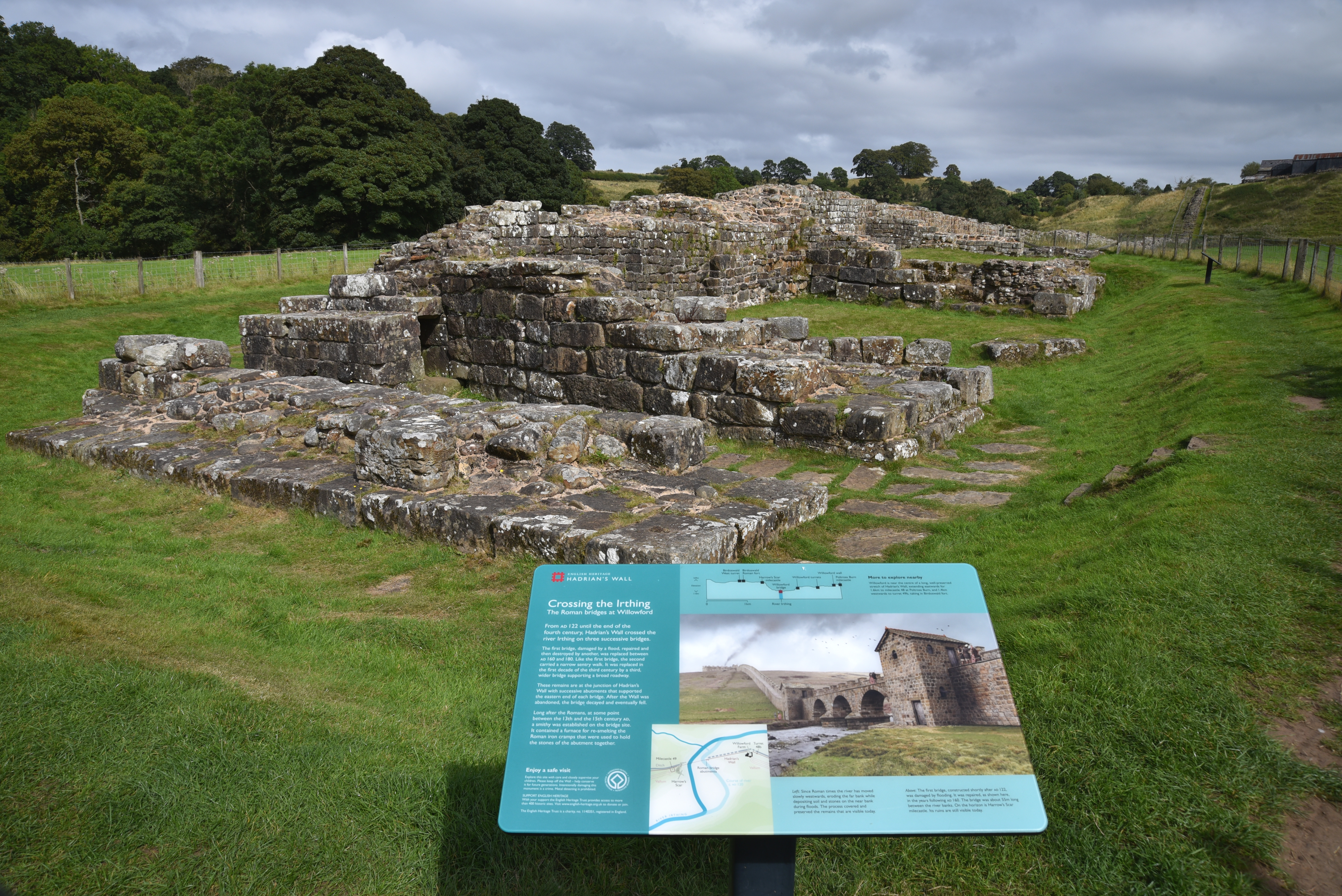A photograph captures the remnants of an ancient stone-built fort, likely one of the many historic sites scattered along Hadrian's Wall. The ruins, constructed from grey stone speckled with white, rest on a verdant grassy platform. Only fragments of the original fortifications remain, with several foundational remains and short sections of wall hinting at the once formidable structure. On the left-hand side of the image, a dense cluster of trees adds depth to the landscape, beneath a sky thick with clouds. A National Trust interpretive sign stands at the forefront, its blue and white design providing a detailed and picturesque representation of what the site might have looked like in its prime, further immersing the viewer in the historical context of the scene.